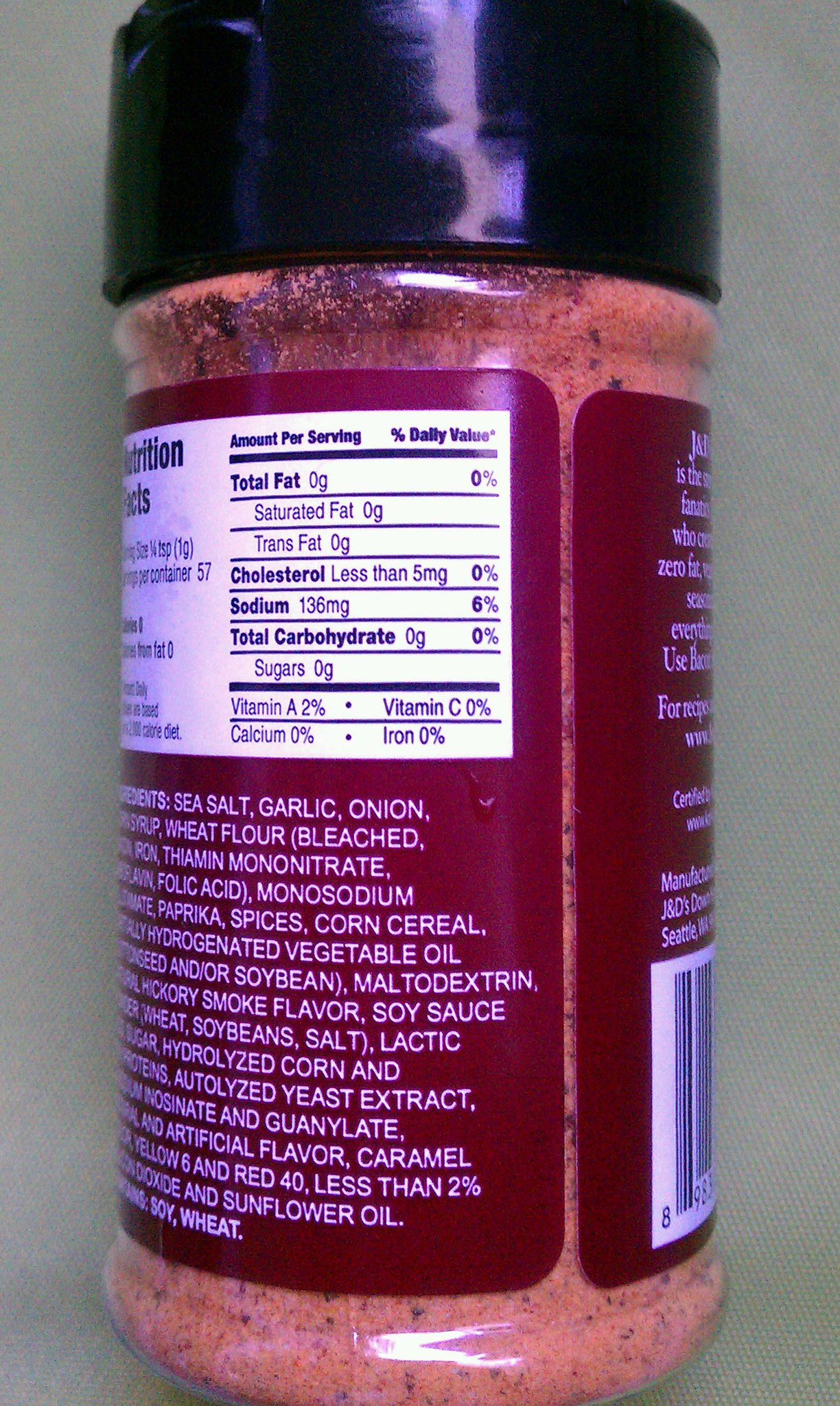The image depicts a close-up view of a cylinder-shaped, transparent plastic canister containing a light pink powdered seasoning with black specks. The bottle has a deep red label with nutritional facts printed in black text on a white background and additional ingredient information in white text on a red background. Key nutritional details visible include total fat at 0 grams, saturated fat at 0 grams, and cholesterol at 0%. The listed ingredients include sea salt, garlic, onion, wheat flour, diamine mononitrate, monosodium something, caramel, less than 2% of Red 40, and lactic acid. The canister is capped with a circular black lid, and it is placed against a gray-black backdrop.